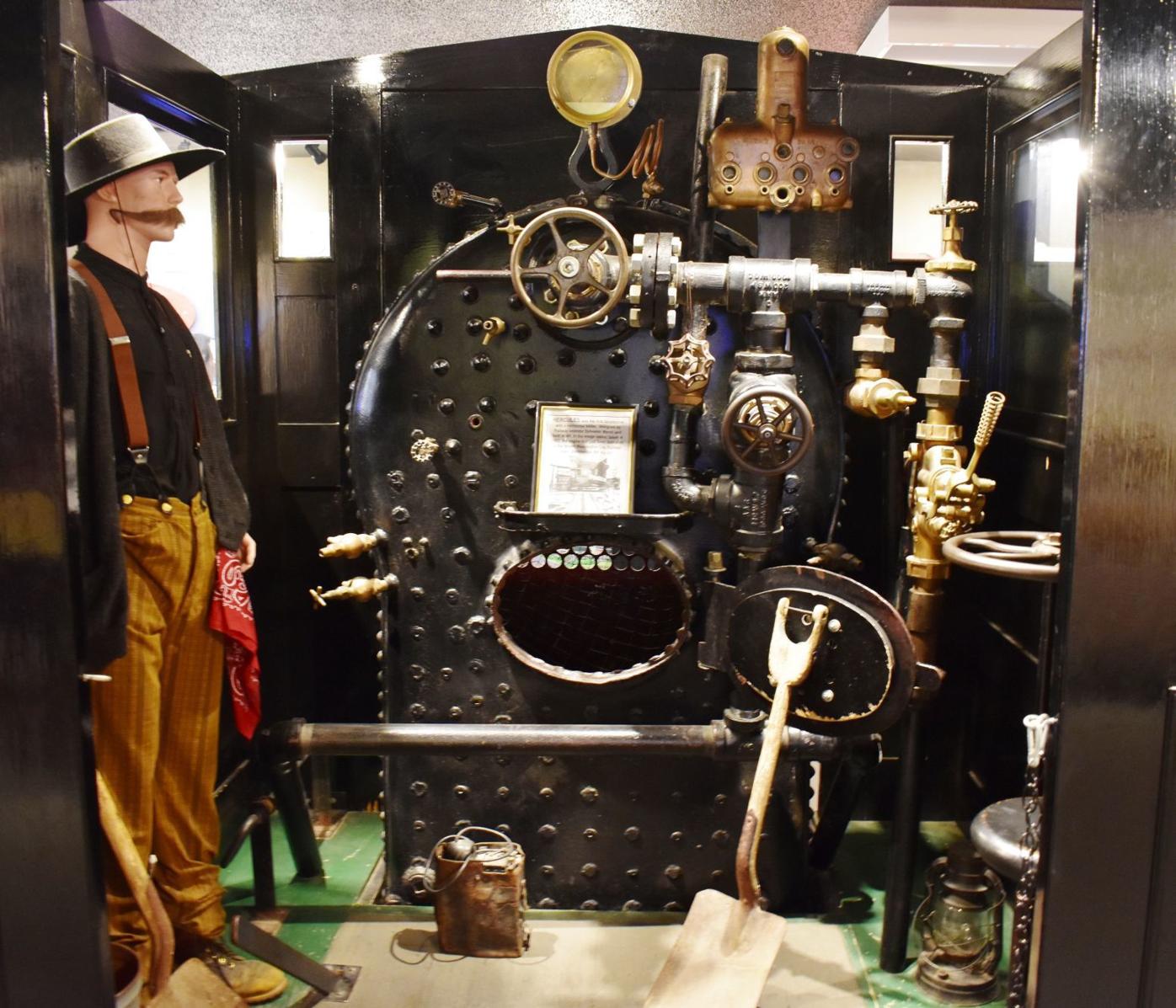This image portrays a detailed historical display, likely from a museum, showing a steam engine room. Dominating the scene is a large, black metal boiler with an open door, revealing where coal would be shoveled inside. A brass wheel sits at the top of the apparatus, surrounded by a complex network of pipes and metallic components made of copper and brass, including a large gauge at the top. A shovel leans against the boiler door, hinting at the manual labor involved, while a small plaque above provides informational context. The room has a green floor and a small box in front of the boiler, with a lantern placed on the ground.

In the background stands a lifelike mannequin dressed in historical workwear: brown pants, black faded work boots, a black button-up shirt, and red suspenders. He also wears a black vest with a red bandana hanging from the front pocket, and a black hat. His prominent mustache and period-accurate attire give a vivid impression of a worker from the age of steam engines. The setting, resembling a part of a steam-powered train or possibly a ship's engine room, vividly captures the industrial atmosphere of the past.